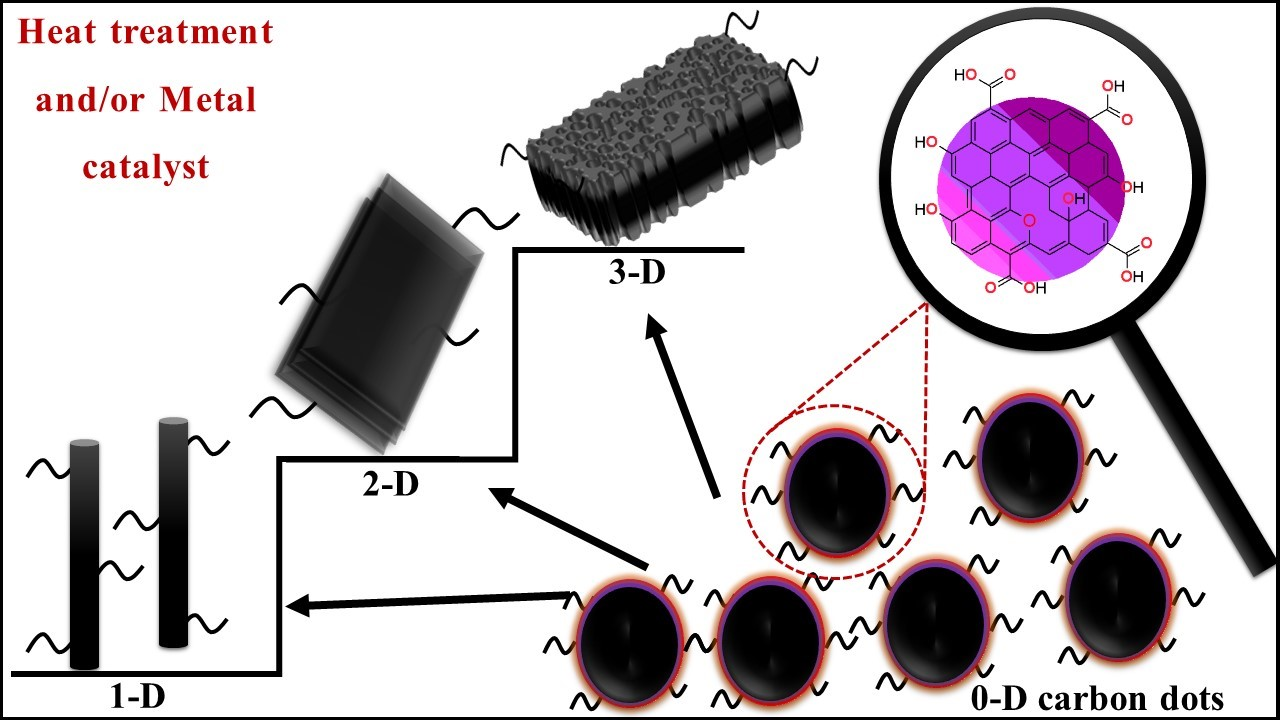The illustration is a detailed scientific diagram depicting the stages of heat treatment and the role of metal catalysts in different dimensions. In the upper left-hand corner, dark red text reads "Heat Treatment and/or Metal Catalyst." The central part of the image features a series of three grey rectangular structures arranged on steps, labeled sequentially from 1D to 3D. The first level, marked 1D, shows two rods with wavy structures on either side. The 2D and 3D levels follow with corresponding more complex structures. At the bottom right, the text "0D carbon dots" is displayed, alongside circular shapes that are magnified within a purple circle, revealing their molecular structure composed of HO, O, and OH. Additionally, a close-up view provided by a magnifying glass highlights the composition of 0D carbon dots, emphasizing the detailed chemical elements involved, such as HONO. The overall theme of the diagram is the scientific breakdown and close-up examination of the catalyst process across various dimensions, from 1D to 0D.